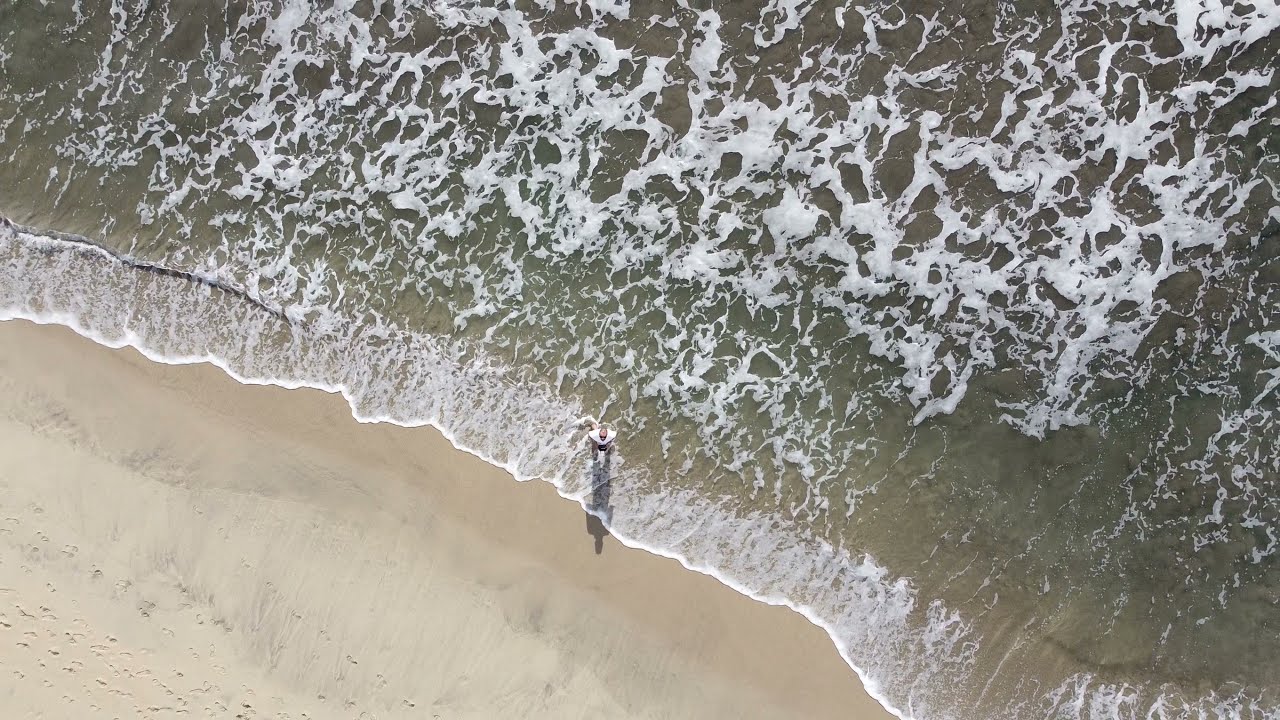This is a horizontal aerial photograph capturing a shoreline scene along an ocean with high waves breaking onto a flat, sandy beach. The image prominently features a person, possibly two, standing at the water's edge where the waves lap against the sand. The sand occupies the bottom left corner of the image, characterized by its fine, white texture, while the rest of the photograph showcases the ocean with its greenish-brown water and white, foamy surf from the crashing waves.

The person, who appears to be controlling a drone as they look skyward, is dressed in a white shirt and situated toward the left side of the image, slightly off-center. They stand in the shallow water, with only their feet getting wet, amidst the clear and somewhat see-through water. The drone, positioned very high up—approximately a hundred feet—captures this serene and dynamic interplay of land and sea.